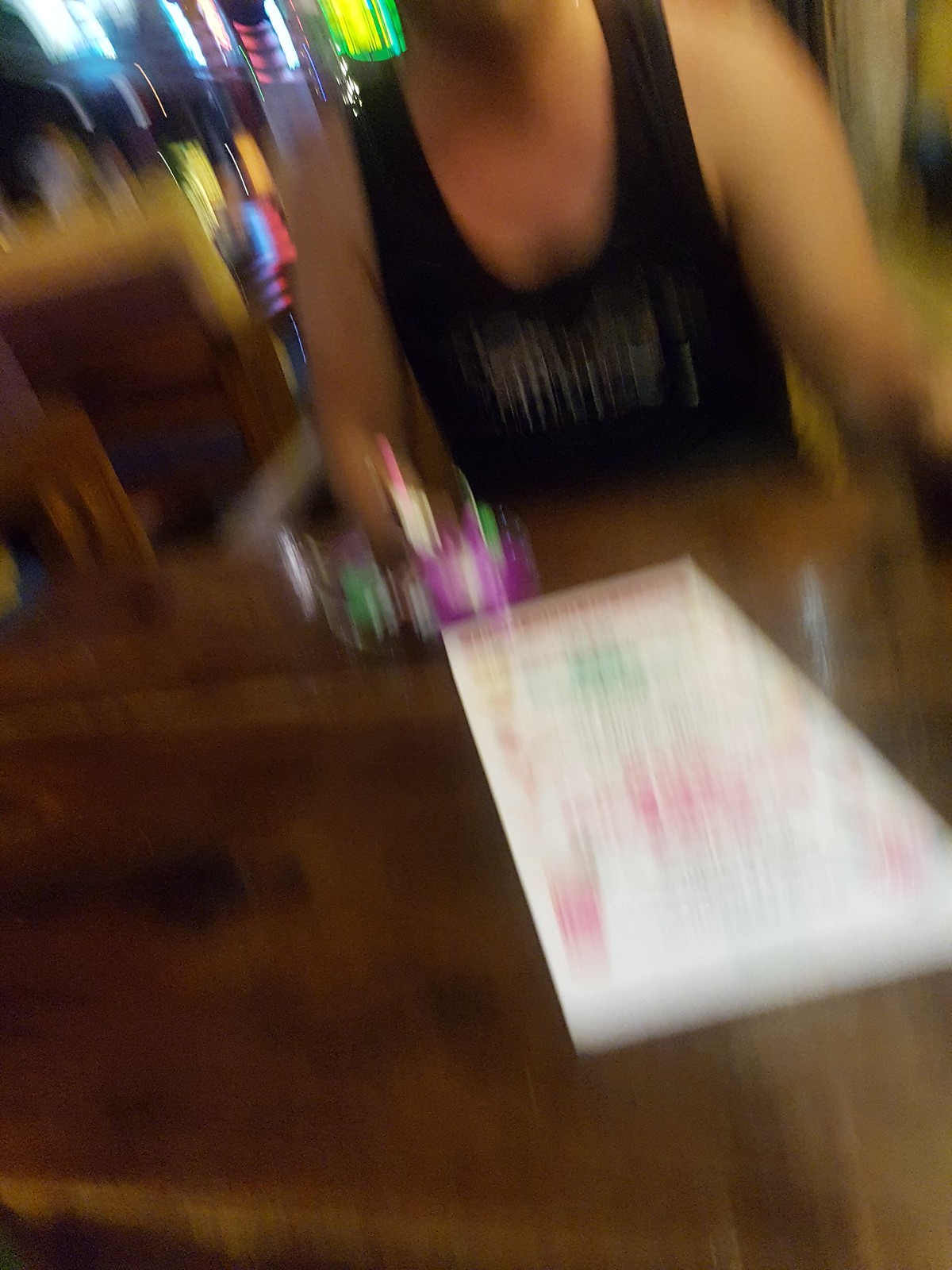In this blurry image taken at what seems to be a bar, a person in a tank top is either serving or enjoying a drink at a table. The beverage in front of them is a striking violet or purple hue, and there are two glasses present. A menu lies on the table, although its orientation is unclear due to the image's blurriness. The setting appears to be in a general seating area rather than directly at the bar. In the background, a table is visible with three or four bottles stacked on it. The table this individual is seated at is a dark brown color, adding to the cozy and intimate atmosphere of the scene. No other people are visible in the frame.